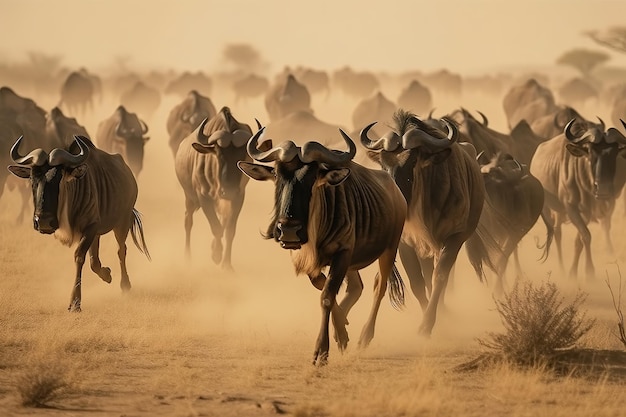The image captures a dynamic scene of a herd of horned animals—likely bison but possibly yaks or antelope—running across a dusty, semi-arid plain. The primary focus is on a few animals near the front and center, showing their large, side-extending horns and long, narrow faces. As they stampede, they kick up clouds of dust, creating a sense of motion and urgency, perhaps fleeing from an unseen threat. The background is filled with more of these animals, fading into a blur, suggesting their number is in the dozens. The dusty ground is dotted with sparse, scrubby shrubs and patches of grass, underlining a dry, late spring or summer setting. The image is characterized by sepia tones, with light and dark browns, grays, and black dominating the color palette, and a hazy outline of trees is visible on the distant horizon.